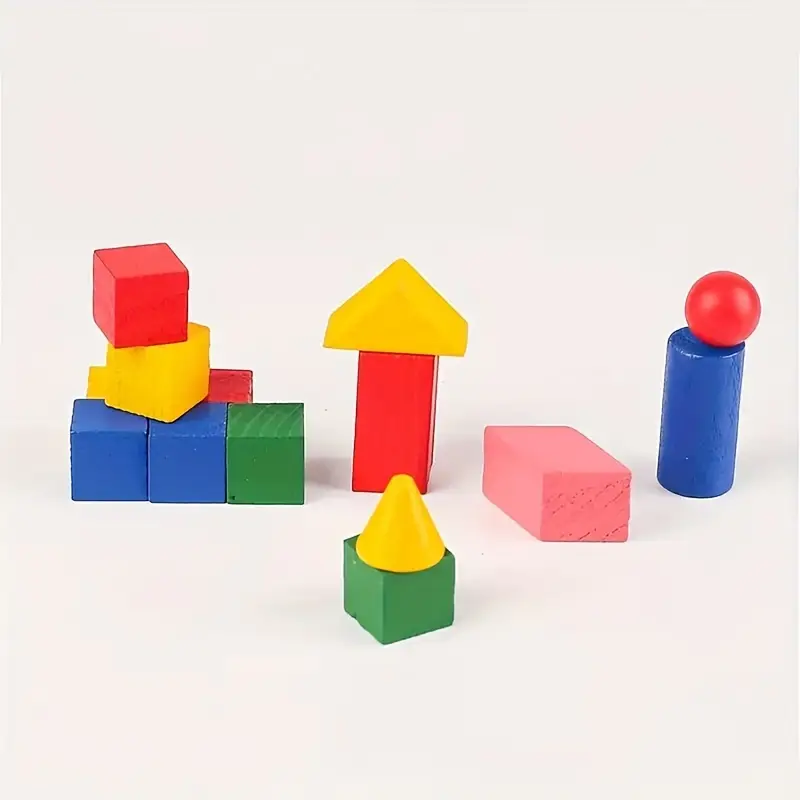This image showcases a vibrant arrangement of children's wooden toy blocks set against a solid white backdrop, drawing the viewer's eyes to the bright, varied colors and shapes of the blocks. Predominantly featuring primary colors such as blue, green, yellow, and red, alongside a lone pink rectangular block, these blocks come in an assortment of shapes including squares, rectangles, triangles, and a single round piece.

On the right side, a tall blue cylinder is topped by a red spherical block, creating a striking vertical structure. Next to it lies the pink rectangle. Moving leftward, a small green square supports a yellow cone. Nearby, a red square stands upright with a yellow triangular block resting on top. The left side of the image displays a more scattered and layered arrangement: two blue blocks, a green block, a red block, and a yellow block lie behind this cluster. At the forefront of this group, a yellow block sits beneath a precariously balanced red block, adding an element of playful instability to the scene. The meticulous yet seemingly random placement of these blocks gives an impression of both spontaneity and careful consideration, embodying the whimsical and exploratory nature of children's play.